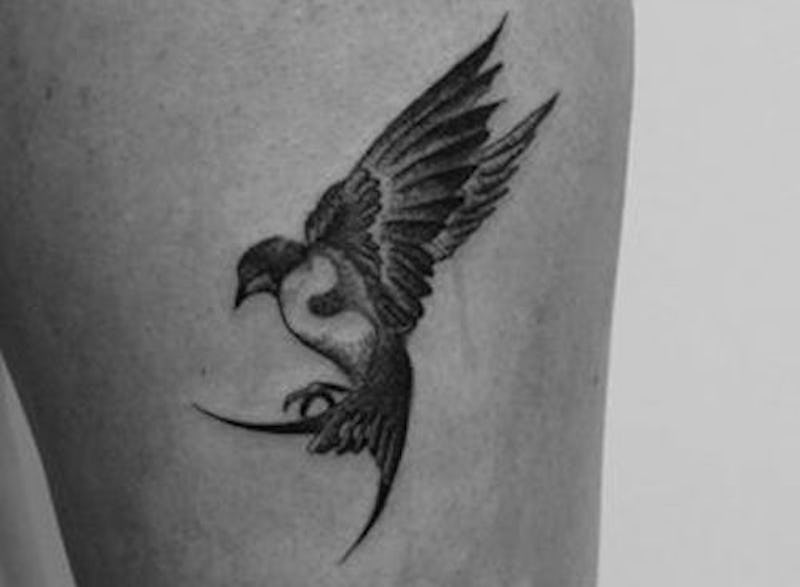This black and white photograph features a detailed close-up of a tattoo on an indistinguishable cylindrical body part, likely an upper arm, shoulder, or upper thigh. The image centers on the tattoo of a tropical bird captured in intricate detail. The bird, seen from its left side, appears to be in mid-flight with its large wings extended upwards as if preparing to land. The tattoo showcases the bird's sharp beak, talons, and elongated tail, all meticulously designed. Although the photo is monochromatic, the bird's features suggest it could be colorful in real life. The background is a light gray, emphasizing the vividness and complexity of the bird tattoo.